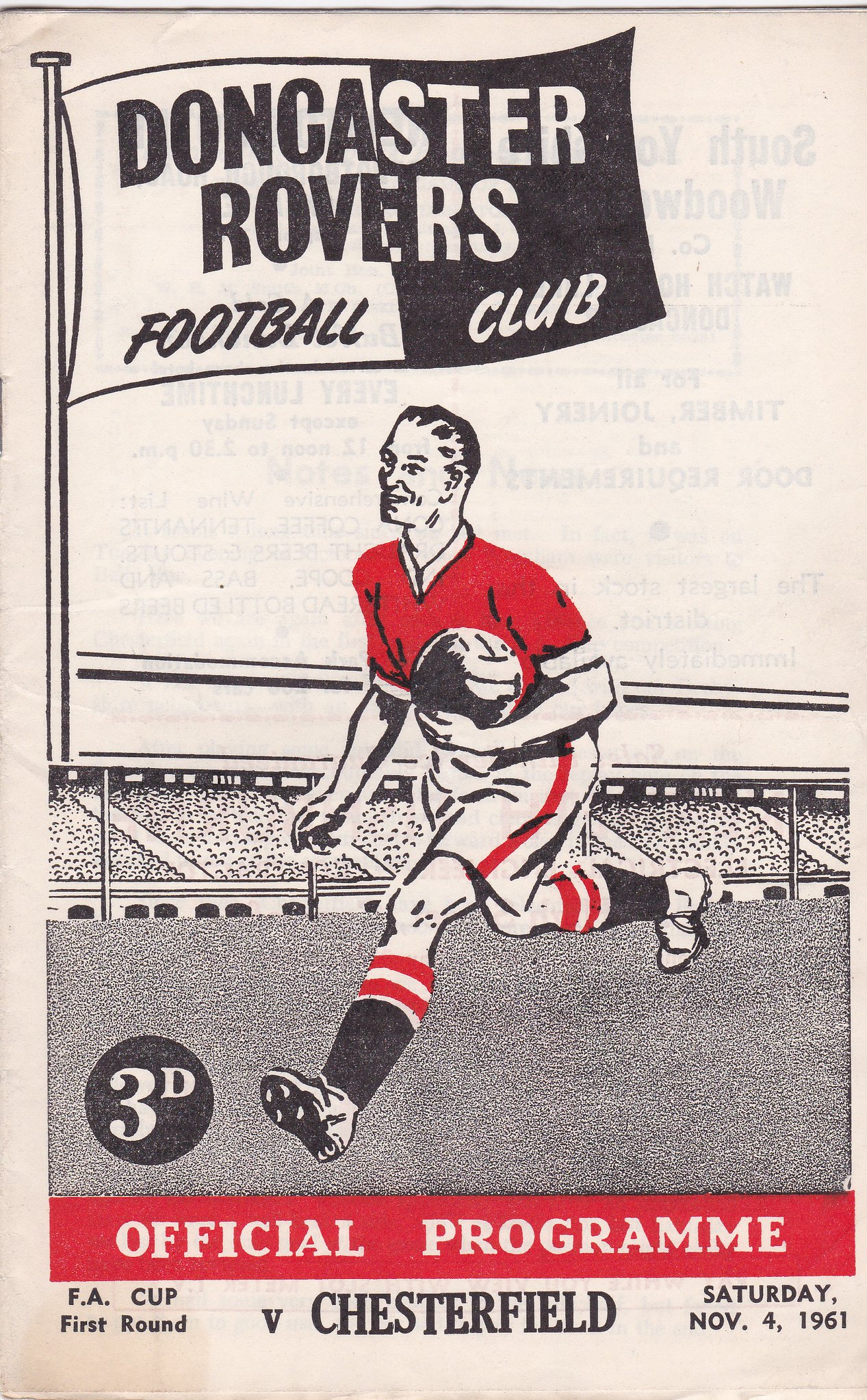This is the front cover of the official program for the Doncaster Rovers Football Club's FA Cup First Round match against Chesterfield on Saturday, November 4th, 1961. The program resembles a paperback newspaper and showcases a vibrant illustration of a soccer player. The player is dressed in a red shirt, white shorts with red stripes, and black and red socks, and shin guards are visible. He is smiling while carrying a soccer ball and running in a stadium filled with spectators. Behind him is a background that includes a black and white flag featuring the Doncaster Rovers Football Club insignia. A prominent 3D circle is also visible, accentuating the official nature of the program. The title "Official Program" is displayed in bold capital letters within a red horizontal bar. Below this, the details of the match are clearly indicated: "FA Cup First Round vs. Chesterfield, Saturday, November 4th, 1961."